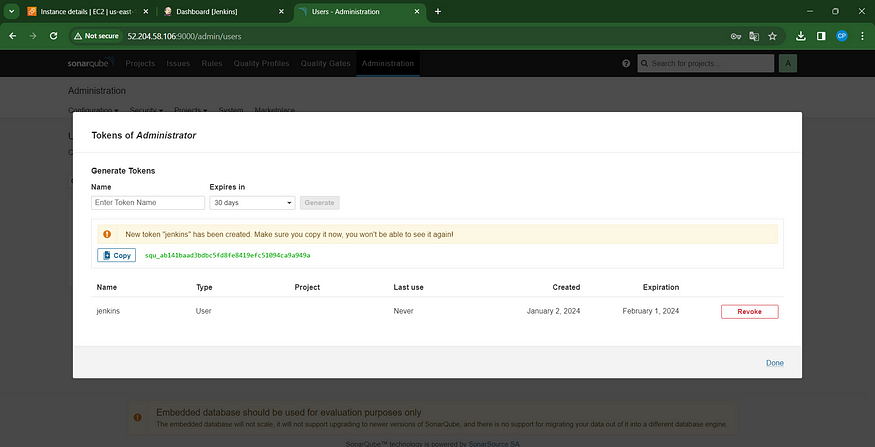This screenshot captures a web page with a dark background, exhibiting a slightly blurry top section, making some text difficult to discern. At the top, there is a series of tabs: "Instance Details," "Dashboard," and "Users Administration," with the "Users Administration" tab being the active one. Below the tabs is an address bar displaying a URL that includes "/admin/users."

Directly underneath the address bar is a black banner featuring several navigation options: "Projects," "Issues," "Rules," "Quality Profiles," and "Administration," with "Administration" being underlined, indicating it is selected. 

The main content of the page is presented in a large white rectangle labeled "Tokens of Administrator." This section provides options to generate tokens. There is a text field labeled "Enter Token Name," and a duration setting titled "Expires In," with "30 days" chosen as the default option. A "Generate" button is available for creating the token.

A notification states, "New Token Jenkins has been created. Make sure you copy it now. You won't be able to see it again." A copy button is provided next to this message.

Further details in the section include:
- Name: Jenkins
- Type: User
- Project: (Blank)
- Last Use: Never
- Created: January 2, 2024
- Expiration: February 1, 2024

Finally, there are options to revoke the token and a "Done" button to complete the process.